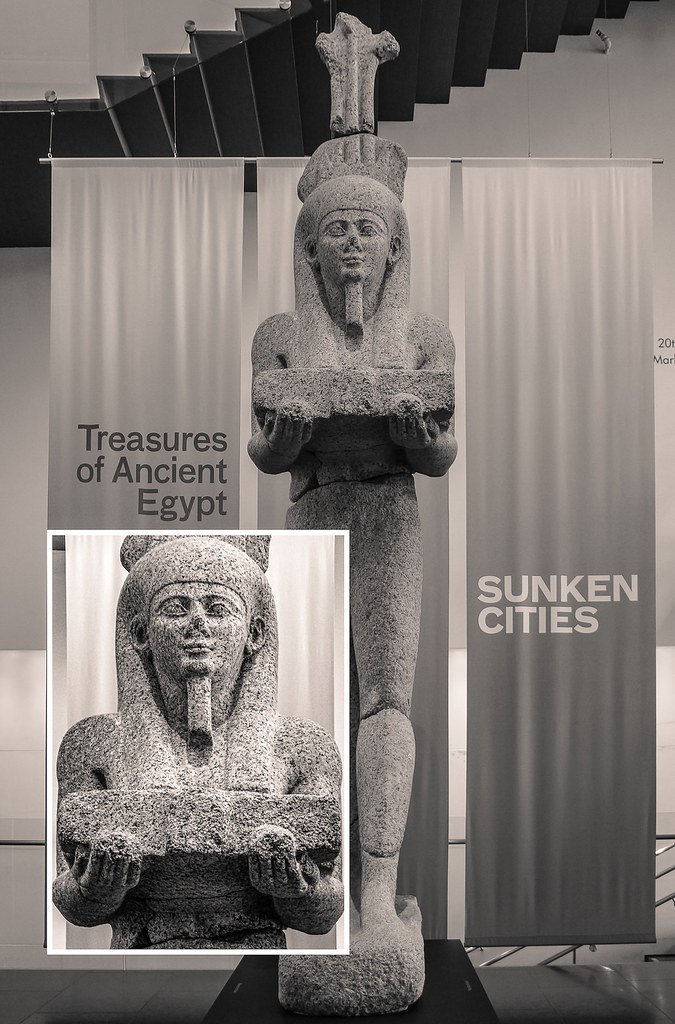The image appears to be a detailed photograph, likely resembling a postcard, showcasing an ancient Egyptian statue exhibit. The central focus is a grainy, black and white statue of an Egyptian figure, adorned with an elaborate headdress that features a cross-like extension at the top and a long, thin beard extending from its chin. The statue, standing erect and facing forward, holds a large tablet or book with both arms outstretched. It rests on a small block base atop a larger black podium-like base. 

The backdrop consists of three vertical banners or curtains hanging from a rod, with visible lines extending upwards and off the top of the image. Behind this setup, black stairs or a similar structure can be faintly seen. Notably, there is a close-up inset of the statue from the waist up, located in a rectangle at the bottom left of the image, partially covering the right leg of the main statue. This inset provides a clearer, more detailed view of the statue's facial features and upper body. 

Text overlays are present on the banners; the left banner bears the inscription “Treasures of Ancient Egypt” in black font, while the right banner displays “Sunken Cities” in white font. The overall composition of the image effectively emphasizes both the statue's intricate details and the thematic representation of ancient Egyptian artifacts.